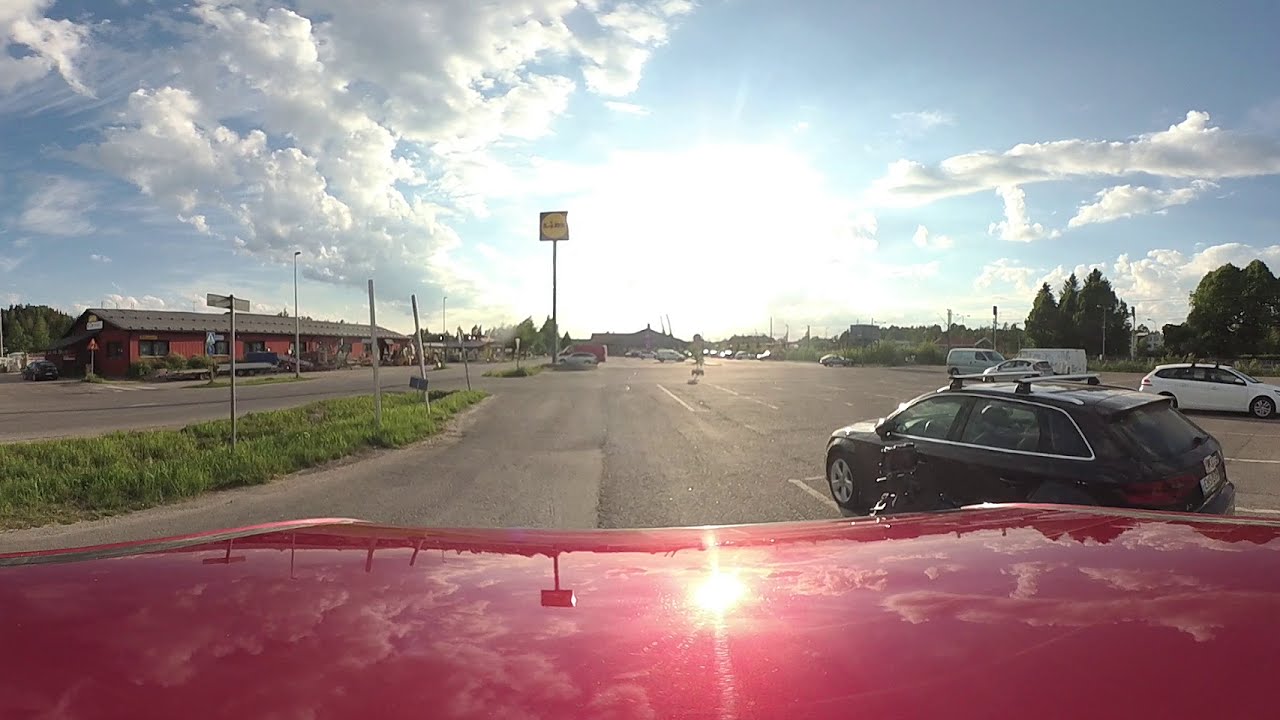The image captures a vibrant daytime scene from the viewpoint of inside a car, showcasing only its reflective red hood. The sun is shining brightly, casting reflections and illuminating a blue sky adorned with fluffy, white and gray clouds, primarily clustered to the left. The car is situated by a spacious parking lot marked by white painted lines on grey asphalt, where various vehicles are parked, including a black hatchback, a white commercial van, and multiple other cars in the distance.

To the left, there's a broad, four-lane road with grassy medians that appears relatively empty at the moment but dotted with a few pedestrians and a couple of vehicles. In the distance, a large red building complex, likely a hotel or motel, stands prominently against the skyline. The scene is lively with the potential presence of restaurants and other buildings, capturing a typical day out, basking in natural light with the sun slightly visible in the far distance.